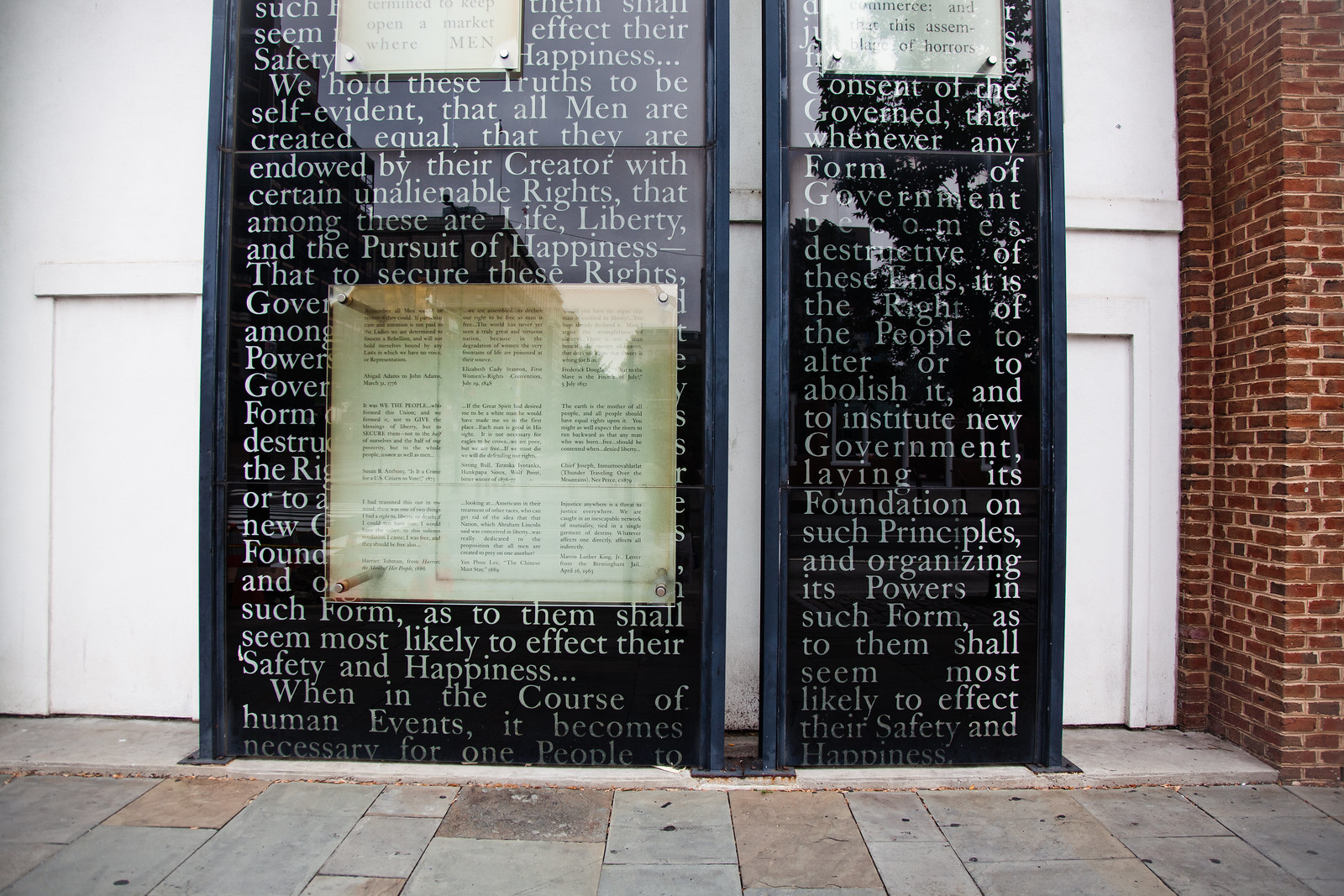The image depicts an outdoor memorial display in front of a red brick building with white wood-paneled recessed walls. The focal points of the memorial are two tall, black display kiosks with glass covers, showcasing important historical texts. The larger kiosk on the left features the United States Declaration of Independence, including a visible second paragraph that reads, "We hold these truths to be self-evident, that all men are created equal, that they are endowed by their Creator with certain unalienable Rights, that among these are Life, Liberty and the pursuit of Happiness." The text is partially obscured by a white piece of paper with additional text in three columns. The smaller, narrower kiosk to the right also contains a historic text, though the details are obscured by another white piece of paper. Both kiosks are situated on a cement-tiled sidewalk with light gray stone tiles arranged in a random pattern, contributing to the dignified and solemn atmosphere of the memorial.